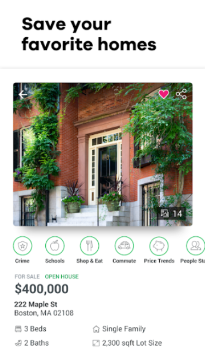A vertically cropped screenshot taken from a mobile application displays detailed real estate information. At the top of the screen, the header reads "Save Your Favorite Homes" in black text on a white background. Below the header, a photograph showcases the exterior of a house, potentially an apartment building, characterized by red brick throughout. The entrance frame is painted yellow, and white cement steps lead up to the doorway. Flanking the entrance are potted plants in cream-colored pots, and lush green vines climb the left side of the building, with a small tree and additional vines on the right side.

Further down, a series of circular icons with light green outlines are displayed against a white background. These icons include a knife and fork, a car silhouette, and a piggy bank, among others. The text beneath each icon, though somewhat blurry, lists categories such as Crime, School, Shop and Eat, Commute, Price Trends, and People SK.

Directly below the icons, small gray text reads "For Sale," accompanied by light green text indicating "Open House." Prominently displayed below that is the bold text "$400,000," followed by the address "222 Maple Street" in bold. The location "Boston, MA 02108" appears in smaller text. The listing details indicate "Three Beds, Two Baths," alongside descriptions noting "Single Family" and "2300 Square Foot Loft size." The entire layout is set against a white background.